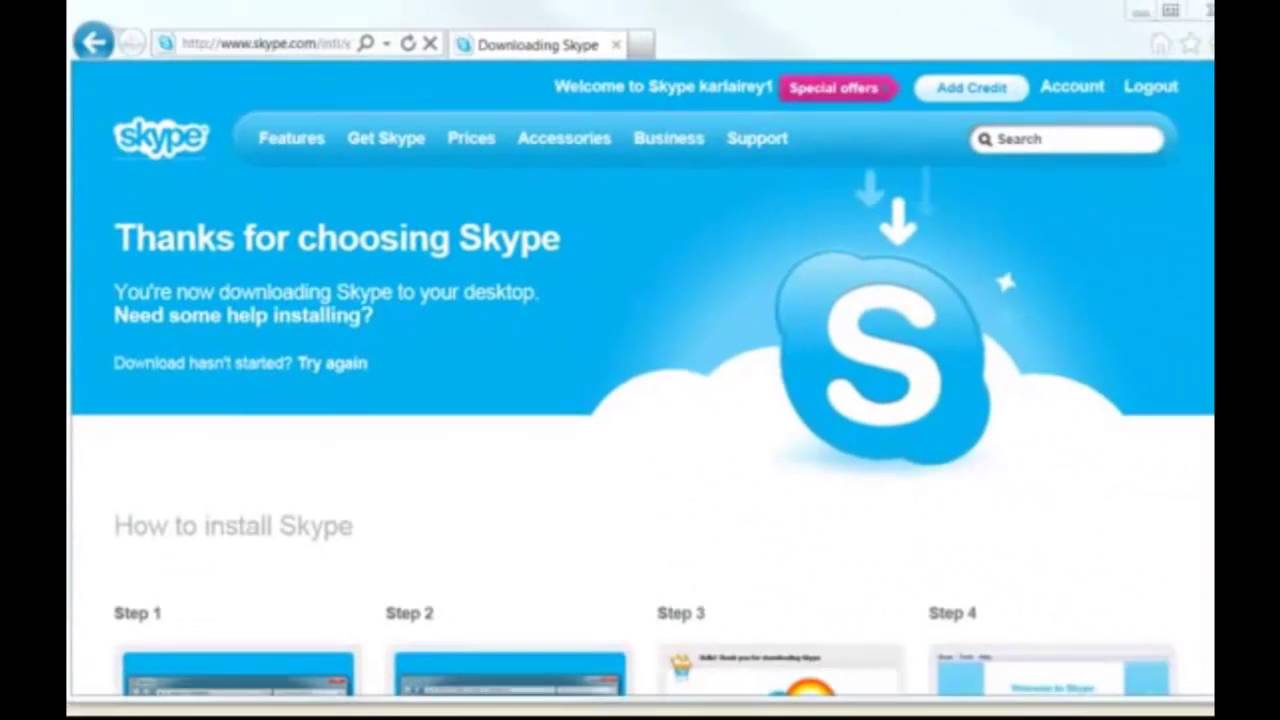This image is a nostalgic snapshot of the Skype website from an earlier era, possibly during the Windows XP days. At the top left, there's a recognizable round back icon in blue, often linked with the Windows XP interface. To the right, a smaller, disabled forward icon in light gray is visible. The URL bar features a mix of light gray and black text displaying `http://www.skype.com`, followed by an unreadable gray forward slash. Adjacent to the URL bar, a magnifying glass with a downward arrow indicates a dropdown menu. Further to the right are refresh and X icons.

The open tab sports the Skype icon on a white background, with a blue logo and a white 'S' signifying the Skype brand. The tab's text in black reads "Downloading Skype." Below this tab is the main website banner, characterized by a deep blue background. On the upper left, the word "Skype" appears in rounded letters, against a cloud that complements the lettering. In bold white text, the banner says "Thanks for choosing Skype." Below, in less prominent white text, it announces, "You're now downloading Skype to your desktop." A highlighted question in bold asks, "Need some help installing?" with a smaller inquiry below, "Download hasn't started?" followed by a bold "Try again."

On the right, part of a white cloud emerges from the blue background. In front of this cloud is a blue circular shape with protruding edges on the top left and bottom right. This shape contains a bubbly white 'S' at its center, reinforcing the Skype identity.